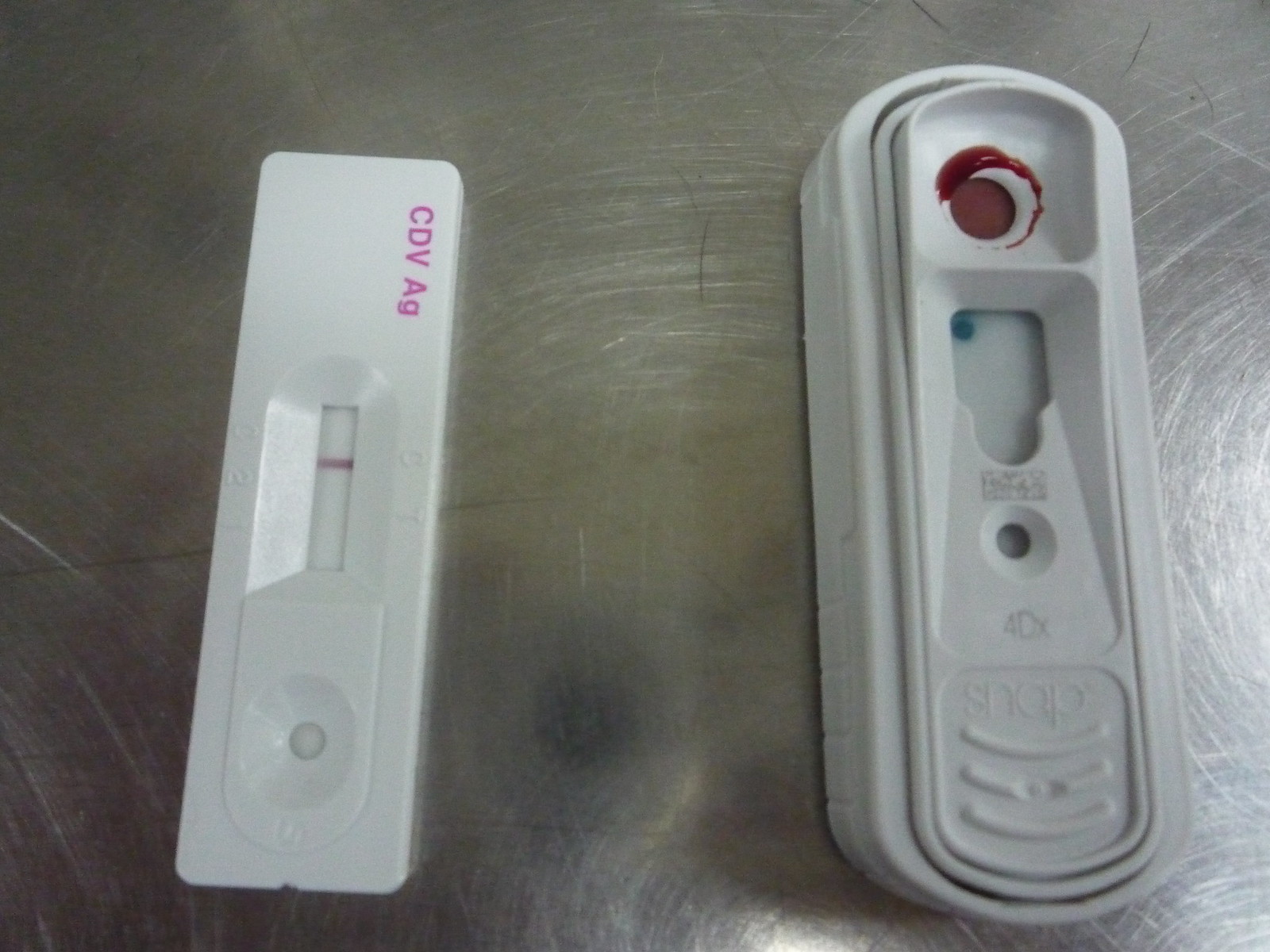On a worn, stainless steel surface bearing the marks of extensive scrubbing, sit two white, rectangular plastic items with curved edges. The first item, positioned to the left, has the text "CDVAG" written in pink. An open section reveals a red strip and some numbers, suggesting it might be a type of medical test. The second item, which is larger and longer, also features an open section, distinguished by a blue circle, indicating it too could be a medical test device. The overall scene is one of utilitarian functionality, underscored by the aged and battered metal surface.